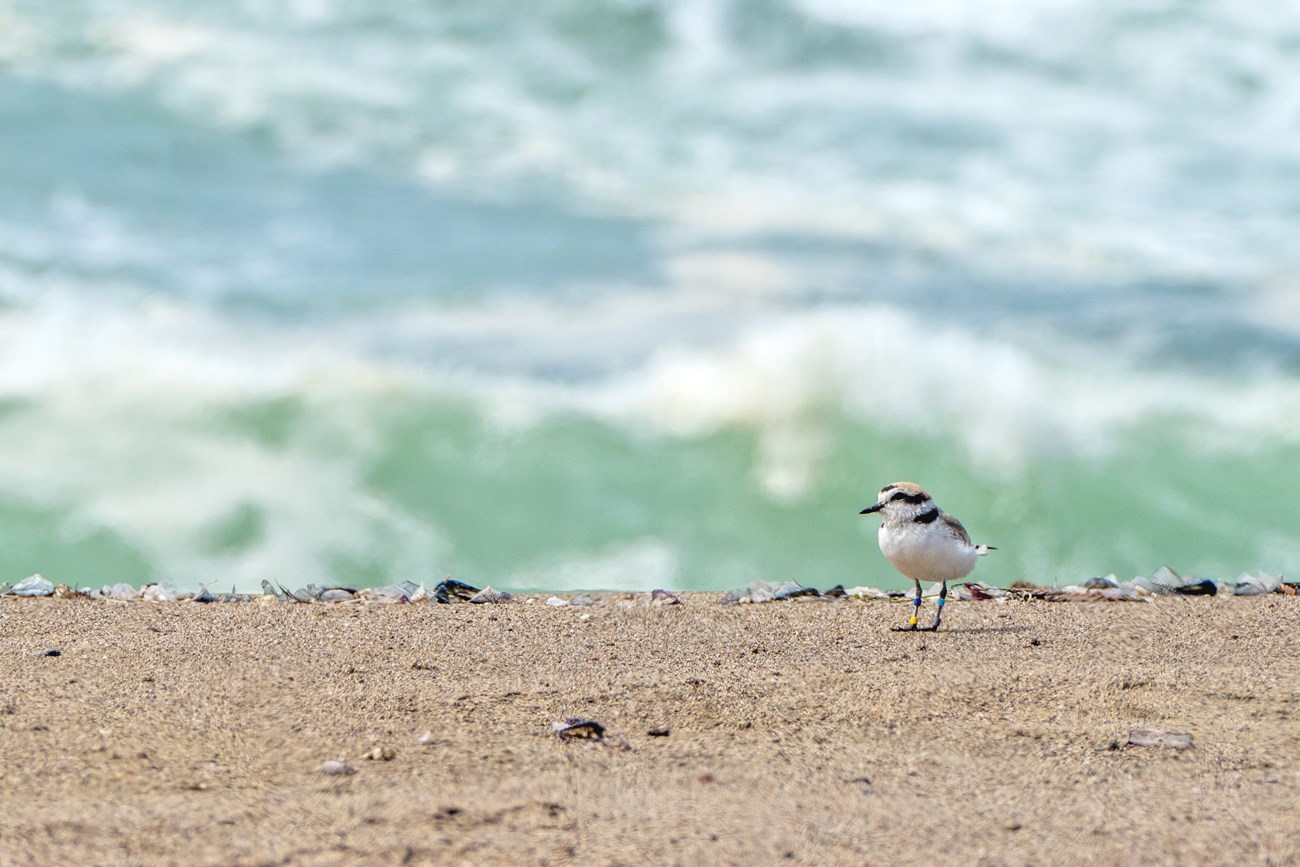A delicate, tiny white bird speckled with black spots stands gracefully on a stretch of light brown sand. This charming creature, identifiable by its slender greenish legs and a petite black beak, appears to be surveying its seaside surroundings. The backdrop features a serene, light green ocean with waves gently crashing ashore, creating a frothy mix of white and blue hues. The sandy foreground is dotted with occasional rocks and individual grains of sand are visible, adding texture and depth to the beach setting.